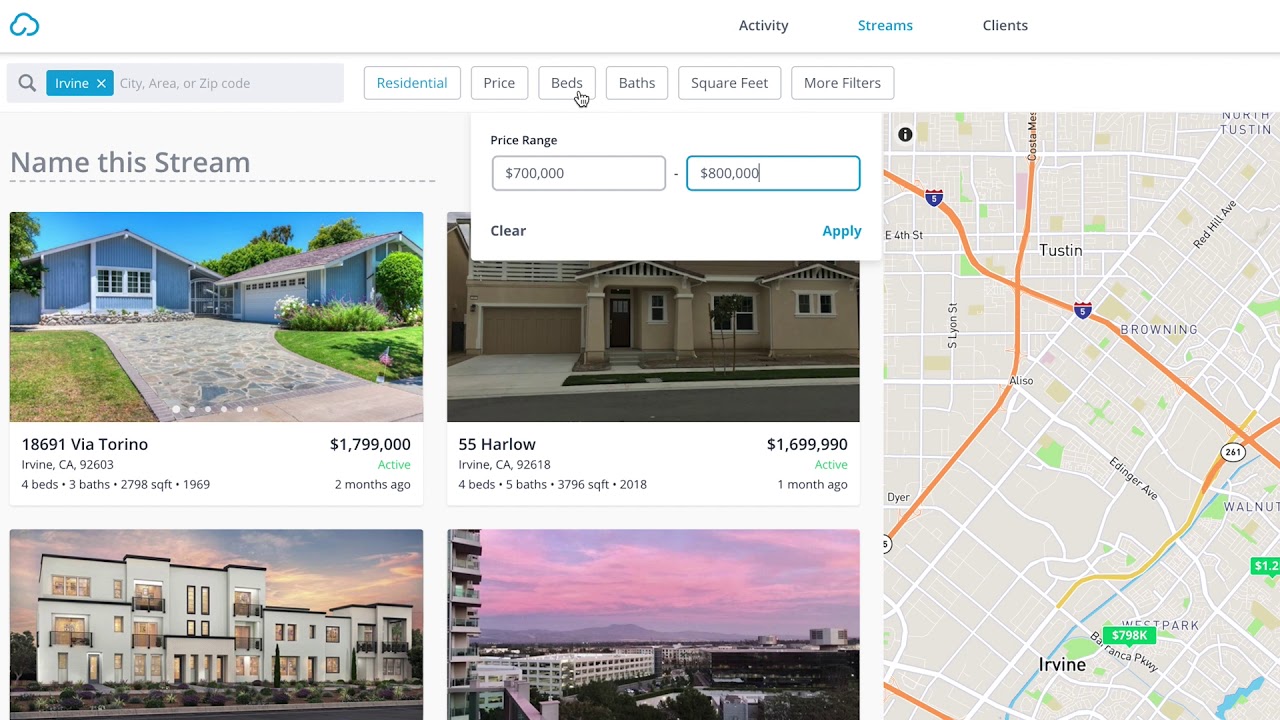The image depicts a real estate website offering homes for sale. At the top of the webpage, there are navigation tabs labeled "Activities," "Streams," and "Clients," with "Streams" highlighted in blue, while the other two are in black. Below these tabs, a search bar allows users to input a city, area, or zip code; it currently displays "Irvine" in white text against a blue background.

Next to the search bar, there are filter options for "Residential," "Price," "Beds," "Bath," "Square Feet," and more. The "Beds" filter is indicated by a hand icon, while "Residential" is active and highlighted in blue. Underneath these filters, the interface prompts users to "Name this stream," accompanied by a dotted line.

The main section of the webpage showcases a price range of $700,000 to $800,000 and displays four property listings, each with accompanying photos and details:

1. A modest blue house located at 18,691 Via Torino, Irvine, CA. It features four bedrooms, three bathrooms, a total of 2,798 square feet, and was built in 1969.
2. A more luxurious property at 55,000 Harlow, also in Irvine, CA. This home includes four bedrooms, five bathrooms, 3,796 square feet of living space, and was constructed in 2018.
3. Another listing highlights a house with a cityscape background featuring pink and purple skies.
4. The final image shows a high-end condominium, possibly beachfront, with a desert-like surrounding landscape.

To the side of these listings, a map provides a geographical visualization of the area.